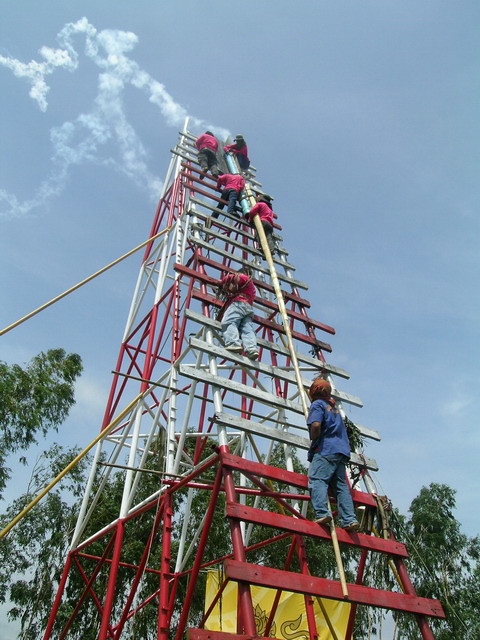This is a color photograph capturing a vibrant scene at a fair or carnival. The image showcases a tall, pyramidal scaffolding structure with a series of alternating red and white steps forming a visually striking pattern. The steps are arranged horizontally and extend upwards, supported by wooden or steel poles that converge towards the top, creating an isosceles triangle shape. Climbing this structure are multiple individuals, predominantly wearing red shirts paired with various colored pants, including light blue, dark blue, black, and gray. One climber sports a gray hat, while the nearest person to the camera is dark-skinned, dressed in a blue T-shirt, blue jeans, and an olive green and red striped scarf. This individual also appears to be barefoot or wearing brown shoes. The vivid scene includes yellow poles that support the structure and a yellow flag adorned with a serpent-like creature fluttering at the top. The background highlights a clear blue sky with faint clouds to the left and a line of tall, dark green trees along the bottom edge of the photo, emphasizing the eventful climb and the festive atmosphere.